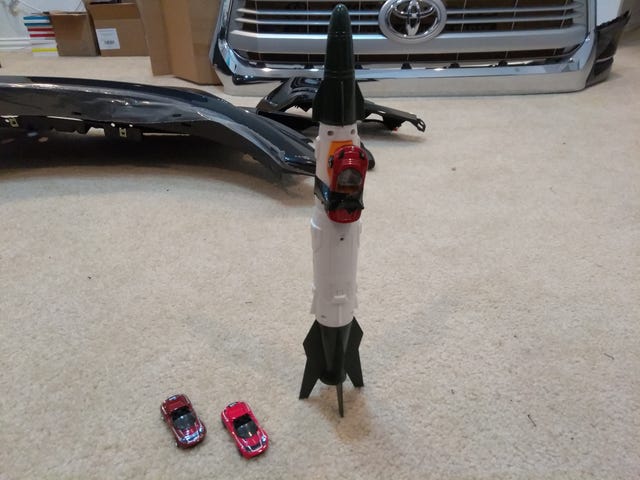The image features an intricately detailed, plastic model rocket with a black nose cone, black fins, and a predominantly white body. Affixed to the rocket with black electrical tape is a red Hot Wheels car. Positioned to the left of the rocket are two similarly sized toy cars: a burgundy convertible and a pink convertible, both angled downward to the right. The scene unfolds on a floor covered in an off-white carpet with speckles, dirt, and scuffs. The backdrop reveals the grill and front bumper of a Toyota vehicle, along with additional car parts, likely dark-colored fenders, and various stacked cardboard boxes in the upper-left corner, suggesting the setting is an interior garage or storage area.